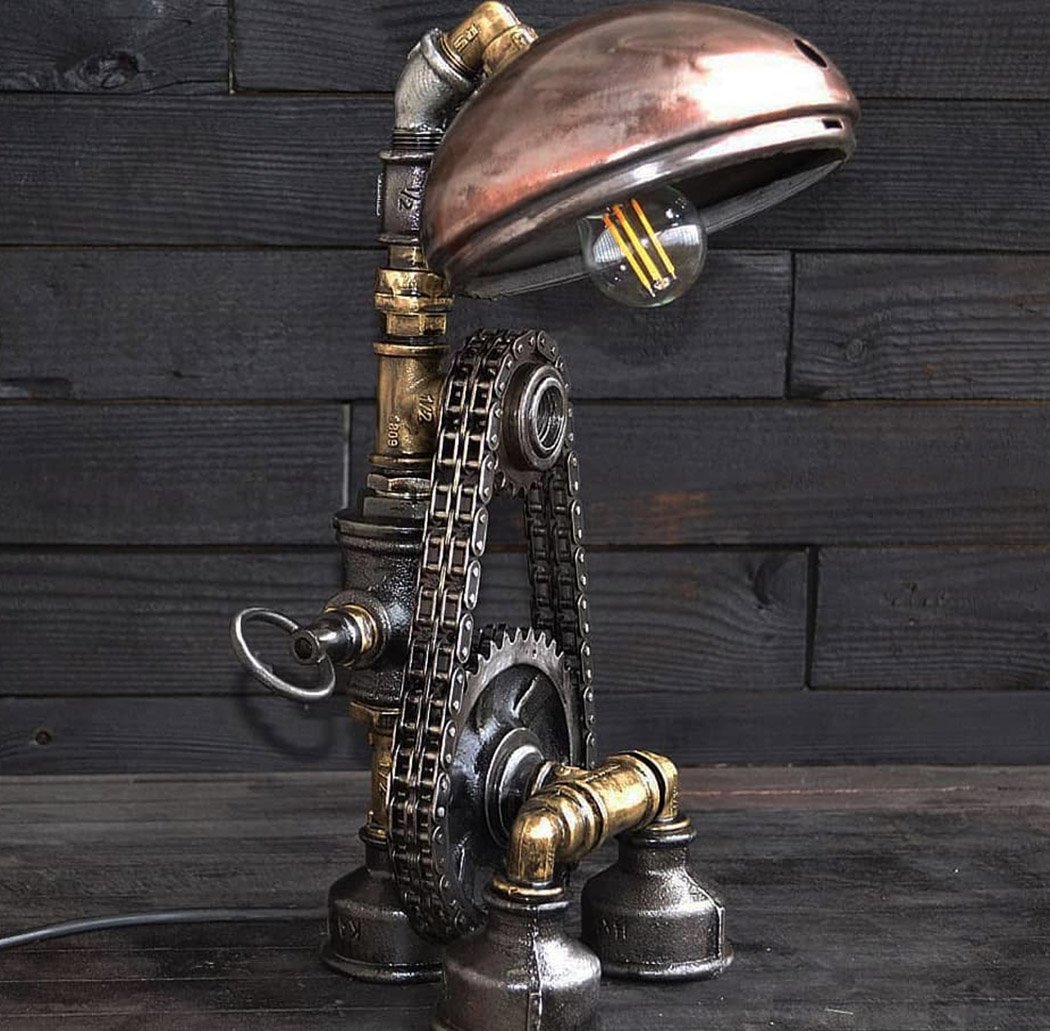The image depicts a highly intricate steampunk-inspired contraption that ostensibly functions as a lamp. Positioned atop a dark, weathered wooden table, the device stands out against a backdrop of dark wooden planks, partially painted in black with patches of unpainted wood. The lamp features a complex structure, consisting of various metal components, including thick iron feet interconnected by brass tubing. Closer to the viewer, these feet are linked to an elaborate system of gears—a large gear connected to a smaller one by a robust double chain. The lamp is adorned with a ring handle on its left side, and an old-fashioned light bulb with three faintly glowing filaments sits at the top, suggesting the lamp is operational. A cord emanates from the left side, arching slightly downward. The entire assembly showcases an eclectic mix of metals, including brass, bronze, steel, and copper, emphasizing its artistic rather than practical nature.